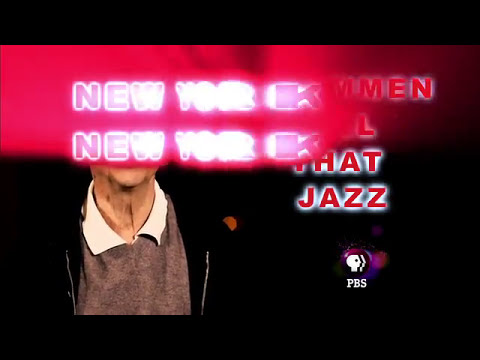The image is a screenshot from a PBS TV channel, featuring an older man with a crepey neck, wearing a white collared shirt underneath a brown sweater vest, and an open black zip-up jacket that blends into the dark background. Horizontal black bars frame the top and bottom of the screen. The man's face is obscured by a red mist effect, allowing only his chin to be visible. Overlapping this effect in glowing white-highlighted red font, it says "New York, New York," with the letters "W" and "Y-O-R" especially emphasized, almost blindingly. Behind these words, additional text in red reads "That Jazz." The PBS logo is displayed in the bottom right corner of the image.